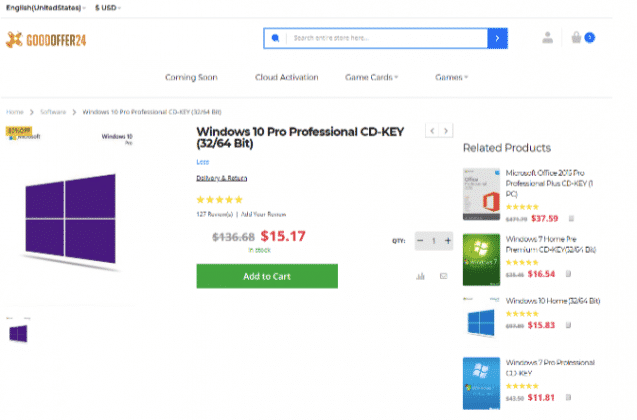In the upper left corner of the image, the text "(English (United States))" is displayed in black, along with a black dollar sign "USD." Below it, an orange or dark yellow airplane symbol is situated next to the text "Good Offer 24." In the middle, within a blue rectangle, there is a search bar containing an arrow pointing to the right, followed by the text "Coming Soon: Cloud Activation Game Cards and Games."

On the left side of the image, there are four large purple squares, which likely represent the Windows operating system. Below these squares, in black text, is the description "Windows 10 Pro Professional CD-key" accompanied by five yellow stars indicating a high rating. The original price "$136.68" is shown struck through, with a discounted price of "$15.17" highlighted in red. A green rectangle with the "Add to Cart" option is located below the price.

On the right side, several related products are displayed with their respective prices in red:
- "Microsoft Office" priced at "$37.59"
- "Windows" priced at "$16.54"
- "Windows 10 Home" priced at "$15.83"
- "Windows Professional" priced at "$11.81"